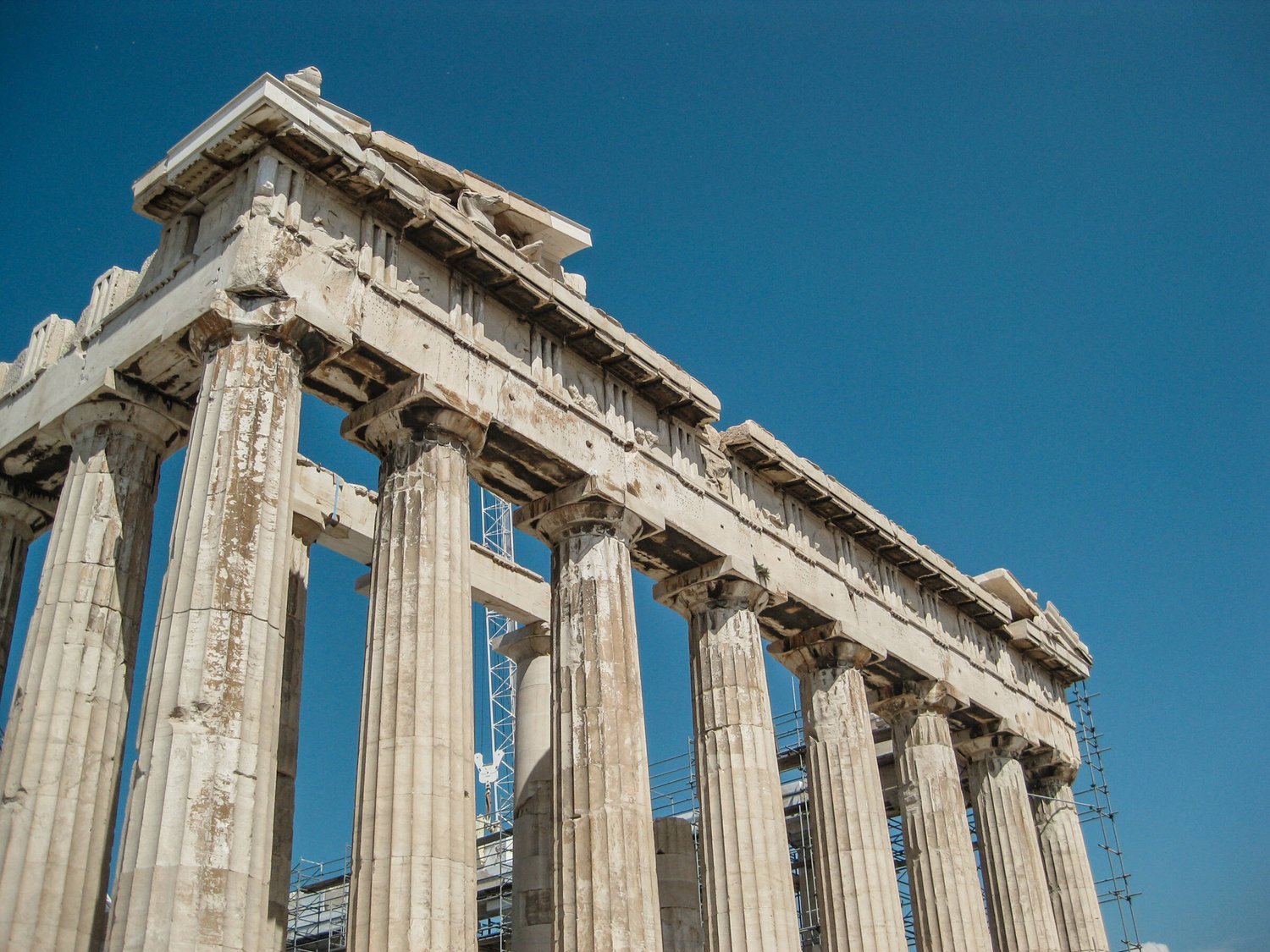This photograph captures an ancient ruin, likely located in Italy or Greece, featuring a series of tall, distressed white to off-white columns reminiscent of Greek architecture. The columns support a stone structure on top, which itself shows signs of decay with missing chunks and chipped corners, exposing a brownish underlayer beneath the faded white paint. The image was taken from a low vantage point, directing the viewer's gaze upward towards the columns and the remnants of the roof, omitting the ground and steps below. In the background, a gradient sky transitions from bright to dark blue, completely cloudless, underlining the age and ruinous state of the structure. Scaffolding is visible near the building, suggesting ongoing restoration efforts. The pristine blue sky, combined with the stark appearance of the columns, creates a striking contrast against the aged architecture.